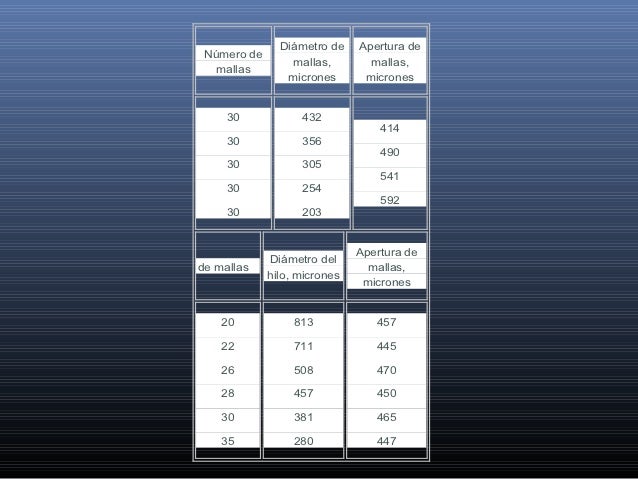The image consists of a background gradient ranging from dark blue at the bottom to light blue at the top. White, thin horizontal lines traverse this gradient backdrop. In the center-left section, a rectangular table is split into six sections—three on the top and three on the bottom. Each section in the table lists data points and headings. The headings and numbers appear to be in a language other than English, possibly Spanish. The headings for the top sections read "numero de males," "diametro de males microns," and "apertura de males microns," followed by various numerical values such as 30, 432, 414, etc. The bottom sections feature similar headings like "de males," "diametro del hilo microns," and "apertura de males microns," with their respective values, including 20, 813, 457, among others. The detailed, organized presentation of the data indicates it might be part of a scientific or technical chart.